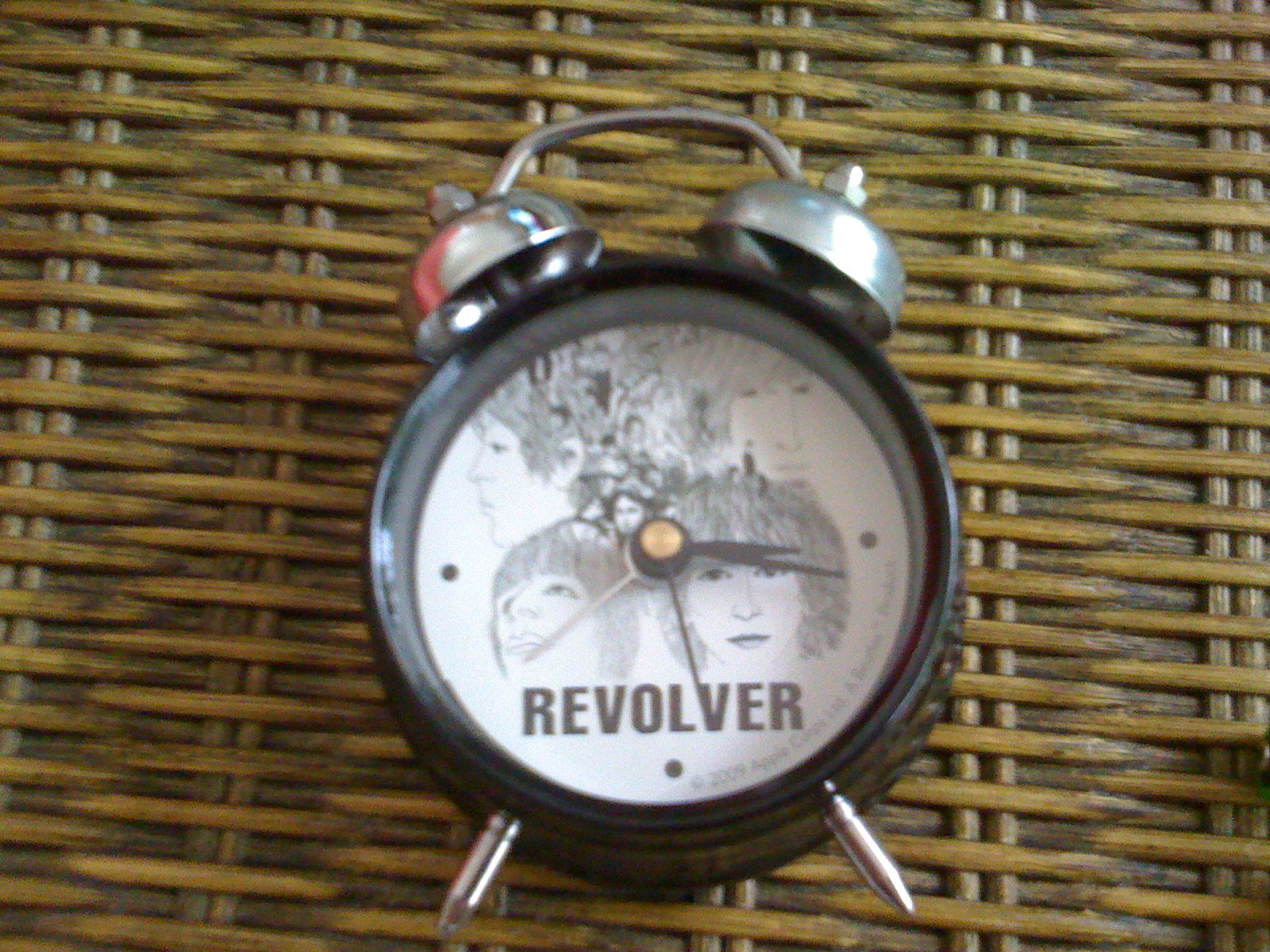The image depicts an old-fashioned alarm clock with a black, circular face, adorned with silver bells on top and two pointed silver legs. The clock has an hour hand, a minute hand, and black and silver markers, but lacks numerical indicators. The face of the clock features the iconic black-and-white artwork from The Beatles' album "Revolver," showcasing detailed sketches of the band members' faces—John, Paul, George, and Ringo. The album title "Revolver" is prominently displayed in block letters at the bottom. The intricate drawings cover the upper portion, with larger faces interspersed with smaller ones. The clock is set against a brown wicker or rattan background, and the photograph has a slightly out-of-focus quality.